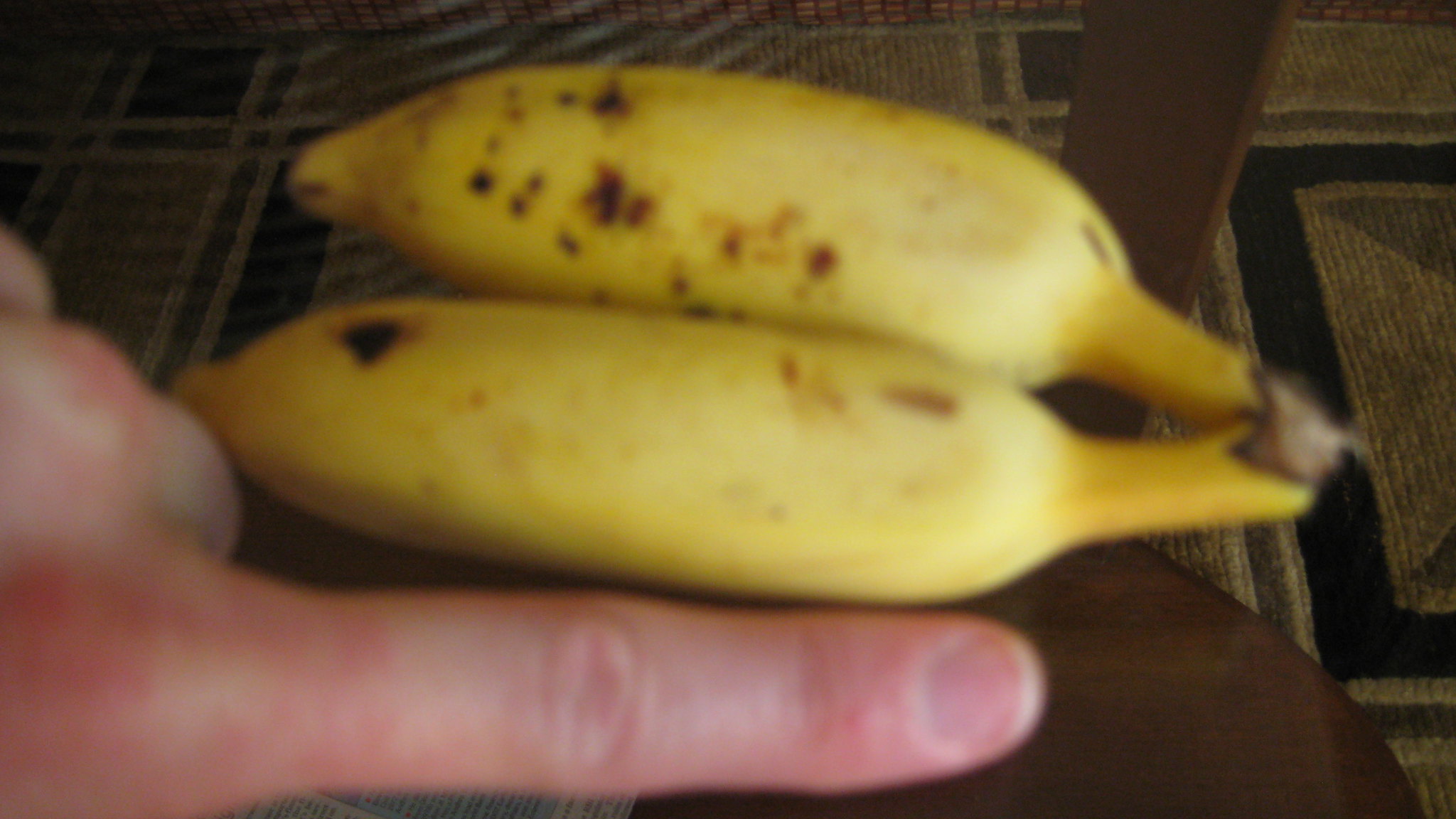The image features two slightly overripe, short bananas, marked with black spots, laying on what appears to be the edge of a brown table. One banana lies completely on the table, while the second banana seems to be balancing on the table’s edge. Adjacent to the bananas, a person’s left hand—with a fair-skinned pointer finger—rests next to one of the bananas, indicating the bananas' short length by comparing it to the length from the finger's tip to the knuckle. The background includes a glimpse of a patterned rug with squares in shades of brown, beige, and black, and possibly a slatted chair, although the specifics are unclear due to the blurred quality of the photo.